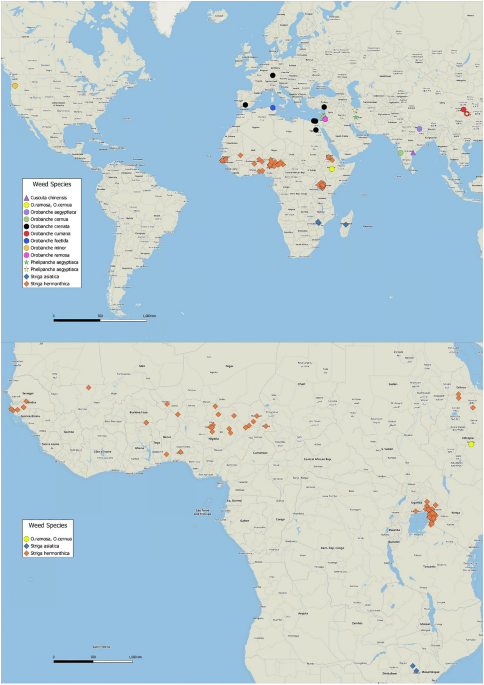The image consists of two separate maps, one of the entire world on the top half and a detailed view of the continent of Africa on the bottom half. The Africa map is selectively focused, showing primarily the western coastline and some parts of the central region, though it excludes the extremes at the north and south. Both maps contain various colored dots indicating something significant, perhaps related to the distribution of weed species, as suggested by the inclusion of a legend on the left side of the world map. The legend lists numerous symbols, including a purple triangle, yellow circle, purple circle, green circle, black circle, red circle, blue circle, orange circle, pink circle, green star, yellow star, blue diamond, and orange diamond, though the corresponding text is too blurry to decipher. Despite the lack of clarity, spots are not densely populated on either map, suggesting a specific study or illustration, which could be useful in an educational or research context. The world map shows distinct concentrations of these dots, such as many orange dots across Africa and scattered black dots in the Middle East and Europe, with occasional blue and pink dots in those regions as well.